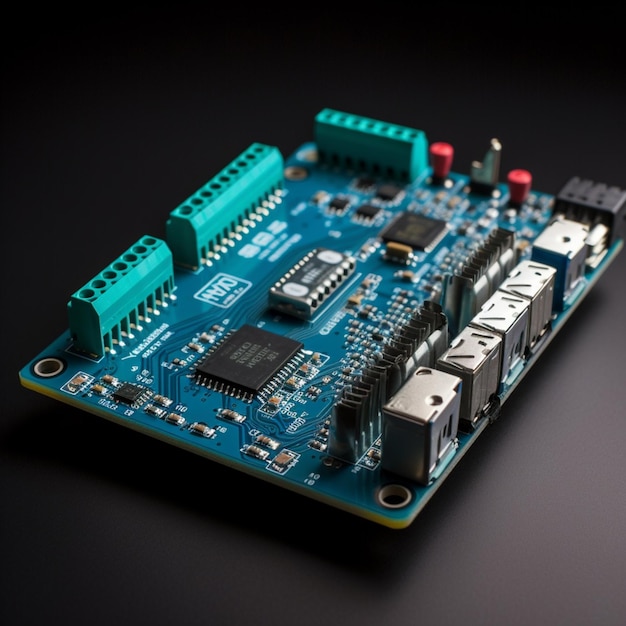This photograph showcases the intricate inner workings of an electronic device, likely a computer motherboard, or possibly a plug-in card or a microcontroller. The green circuit board spans the image, populated with various components. Strikingly, three oblong turquoise-colored components are mounted along one edge, adjacent to five silver-colored square components plugged into the board. A flat, green battery is central to the layout, interspersed with numerous circuits, copper traces, and a multitude of small, precise elements. Red dials and buttons add to the board's complexity, situated near the top edge. On the right, there are metal boxes potentially housing connectors for RJ11 cords or similar interfaces. Additionally, the board features green surface-mounted connectors on the left and top edges, possibly for inputs or outputs. Central to the image are prominent microchips, including two PLCC modules and another central microchip in a socket. Finally, red power attachment terminals are visible at the top right, attesting to the board's multifunctional design.